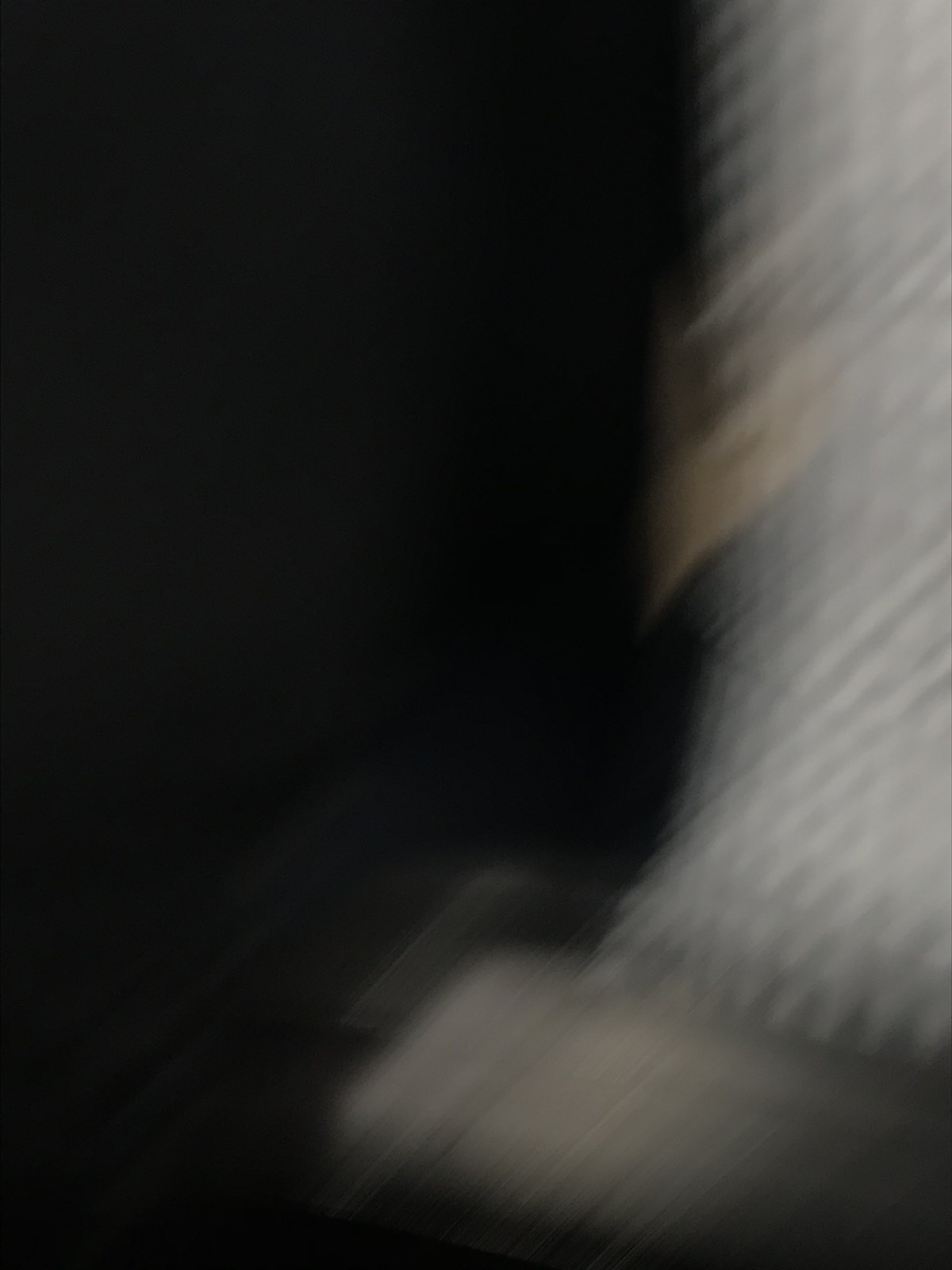The black and white photograph is vertically aligned in portrait mode, featuring a stark contrast between the predominantly black left side and the lighter right side. The right side showcases an indistinguishable blur or smear of white and light gray, interspersed with black dots, giving it a textured appearance. This region may suggest the end of a curved piece of cloth, perhaps resembling a shirt sleeve. The black transitions into dark gray, medium gray, and then to lighter gray shades at the edge, creating a layered effect. Certain areas beneath and adjacent to this blurred material exhibit a diagonal cut texture, further adding complexity to the image. Despite the overall blurriness and lack of clear detail, the interplay of light and shadow suggests a dynamic composition.